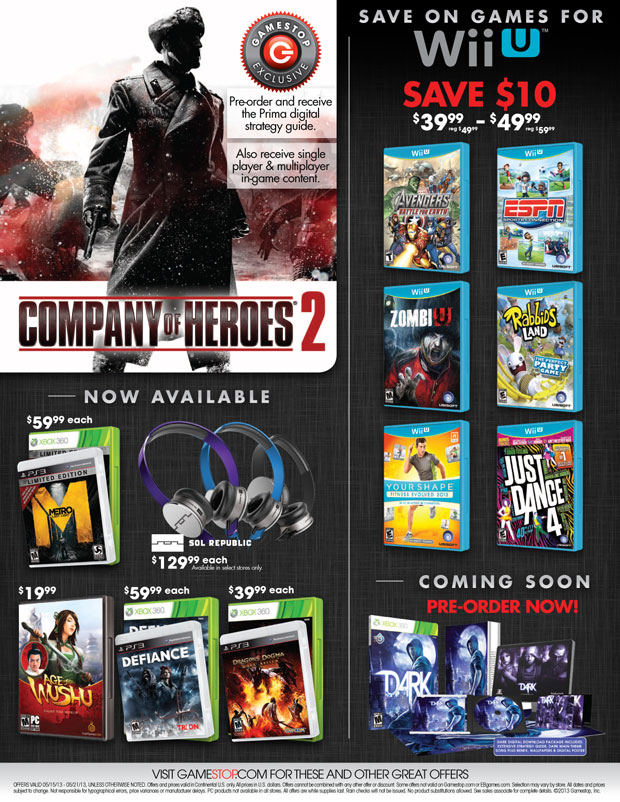In this image, an advertisement from GameStop is prominently displayed, showcasing a diverse selection of video games and gaming accessories. At the top left, the featured video game is "Company of Heroes 2," which has a striking cover depicting a soldier armed with a rifle. Below this, a variety of other video game titles are arranged, including "The Avengers," "ESPN," "Just Dance 4," and "Your Shape," among others. These games are available for different consoles, notably the Xbox 360 and the Nintendo Wii.

Interspersed among the video games are three pairs of headphones, adding to the array of gaming gear on offer. The advertised prices for the video games range from $39.99 to $49.99, while the headphones are listed at $129.99. 

The bottom of the advertisement features a call to action, urging viewers to visit GameStop.com for more great offers. While it seems that this image was taken from the GameStop website, the primary focus remains the diverse selection of video games and the competitive pricing presented in the advertisement.